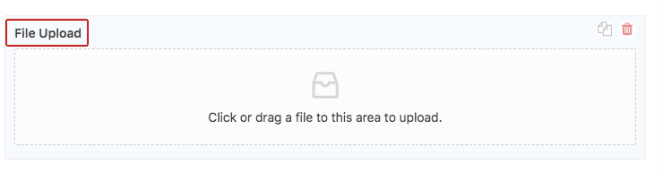In the top left corner of the image, there is a clearly marked file upload section outlined in red. To the immediate right, a small red trash can icon indicates the option to delete uploaded files. Adjacent to it is a copy button, represented by two overlapping document icons with folded corners, indicating the ability to duplicate files.

Centered on the page, there appears to be a filing cabinet icon, possibly representing storage or organization. Below it, there's a directive text with a file emoji: "Click or drag a file to this area to upload." This area is surrounded by a dotted border, forming a large white rectangular box that spans from just below the file upload section to underneath the copy button, offering ample space for file management.

The entire section is accentuated by lighter blue borders around the file upload and copy buttons, providing a distinct visual separation. The "file upload" text is bold and darker compared to the smaller, non-bolded "click or drag" text, which guides users through the process.